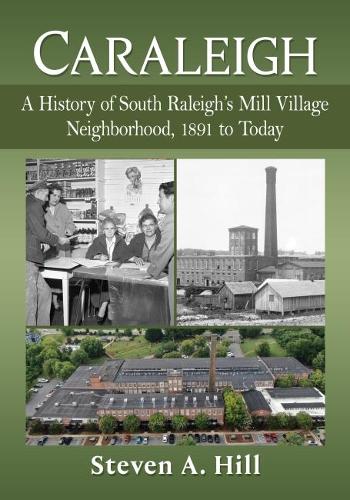The image depicts a green book cover titled "Carolee: A History of South Raleigh's Mill Village Neighborhood, 1891 to Today" by Stephen A. Hill. The cover features three distinct images that narrate the evolution of the neighborhood. The top left image is a black and white photo showing a group of men and women engaged in a discussion, likely around a desk. The top right image depicts a historical factory building with a large tower, captured in black and white, representing the industrial era of the late 1800s. The bottom image offers a contemporary bird's-eye view of the neighborhood, showcasing a collection of houses, greenery, and land. Together, these images underscore the transformation and historical significance of the South Raleigh's Mill Village neighborhood.